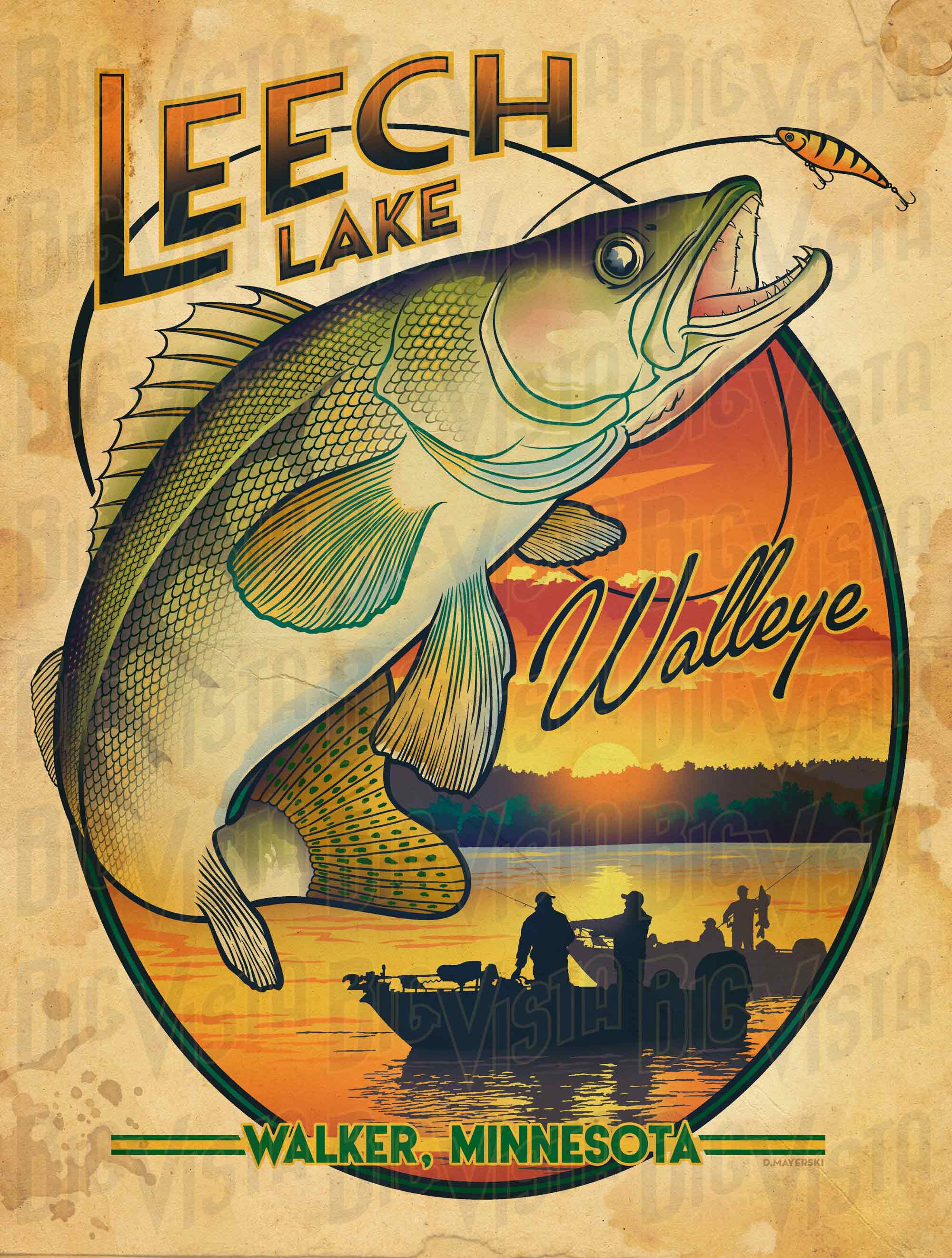This evocative poster advertising Leech Lake and Walker, Minnesota features a detailed and vibrant illustration rather than a photograph. Dominating the scene is a large, vividly colored fish with greenish scales, transitioning to gray towards its belly, and notable pink cheeks. Above the fish, a fishing line dangles a smaller, baited fish, hinting at a narrative of a recent catch. The fish illustration is central, suggesting it's likely a walleye, given the accompanying text.

The poster's title, "Leech Lake," is prominently displayed in the upper left, rendered in striking all-capital letters with an orange-to-black gradient. The word "walleye" appears diagonally in a stylized script font near the middle right, while "Walker, Minnesota" is written in a classic sans-serif font at the bottom in green letters, underscored by a green and yellow line.

In the background, a picturesque scene unfolds with a setting sun casting an orange glow across the sky, adorned with matching clouds. Silhouetted black trees and boats populate the horizon, with one boat prominently featuring fishermen. The scene is encapsulated in an oblong frame, suggesting a sense of depth and immersion. The overall backdrop of the poster is textured with a grunge paper effect, adding a touch of rustic charm and invoking the timeless allure of fishing adventures at Leech Lake.